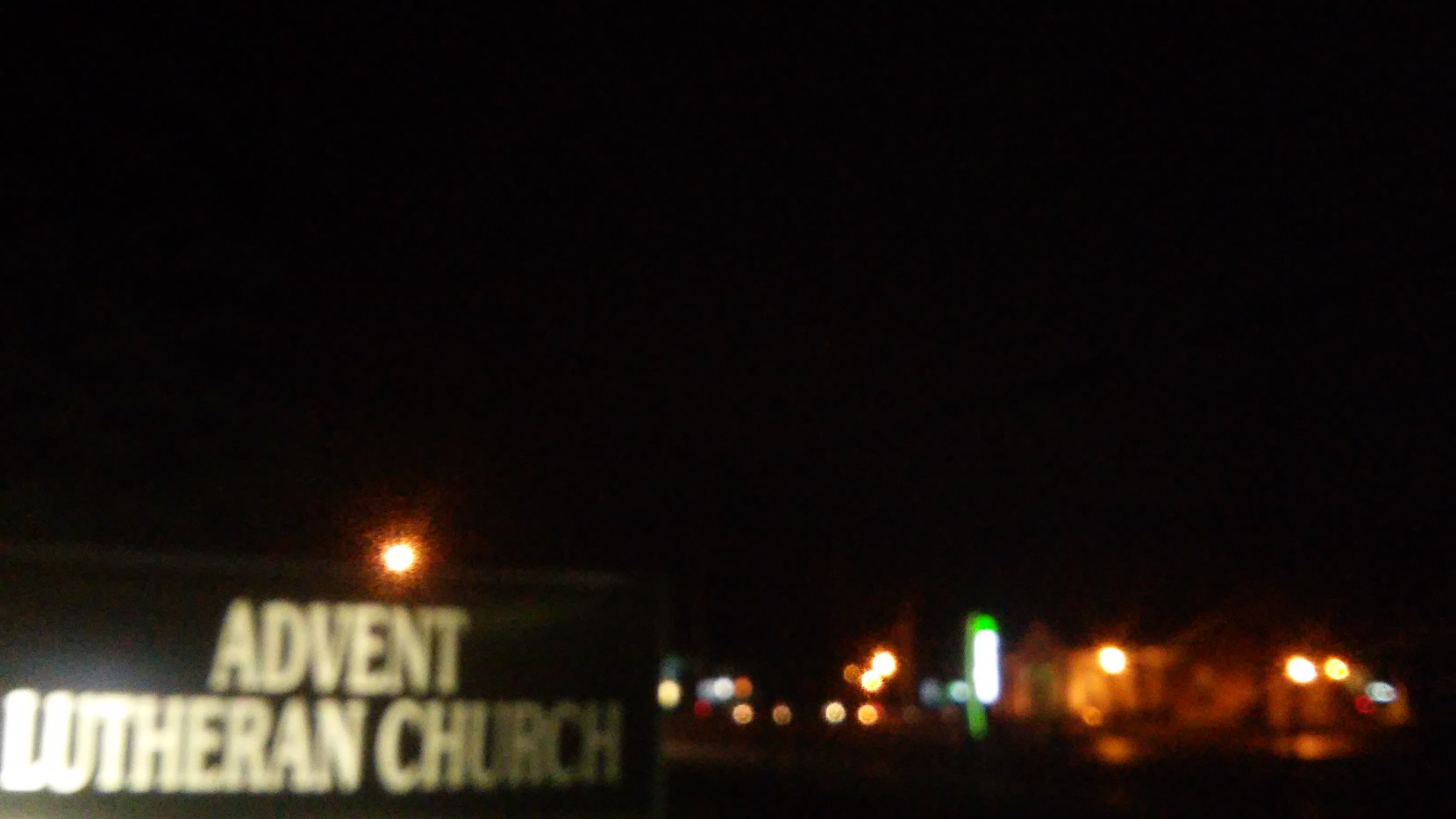This nighttime photograph captures a scene with a predominantly black sky, likely contributing to its blurry appearance. On the left side of the image, an illuminated sign reading "Advent Lutheran Church" stands out prominently. The illumination is stronger on the left side of the sign and gradually fades as it moves rightwards. Above the sign, specifically above the letter "N" in "Advent," there's a reddish-orange light visible in the distance. Towards the right side of the photo, a collection of distant lights, possibly from a small-town skyline or buildings across the street, are visible. Among these lights, a vertical green sign catches the eye, accompanied by white lighting around it.